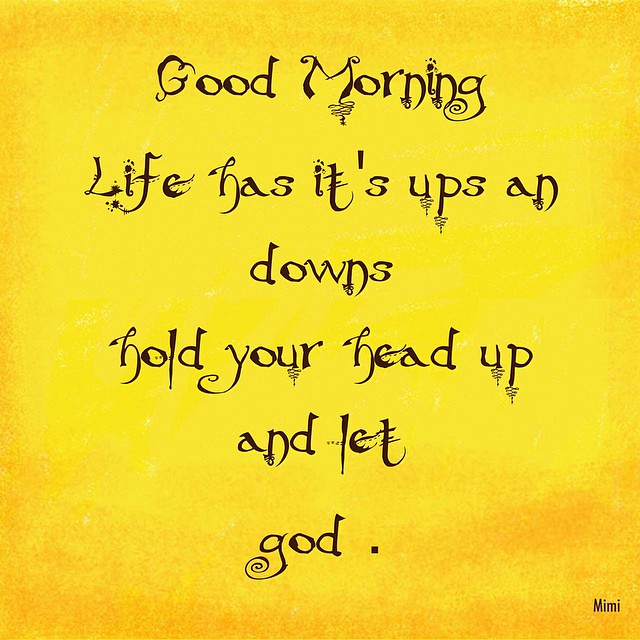The image features a nearly square poster with a bright yellow background and subtle hints of light brown around the edges. Prominently displayed in a unique, decorative font that includes squiggles and curlicues, the text reads: "Good Morning" on the first line, followed by "Life has its ups" on the second line, "and downs" on the third line, "Hold your head up" on the fourth line, "and let" on the fifth line, and "God." on the sixth line. All text is printed in brown. In the bottom right-hand corner, the name "Mimi" is discreetly printed with the first "M" capitalized and the remaining letters in lowercase, adding a personal touch to the inspirational message.